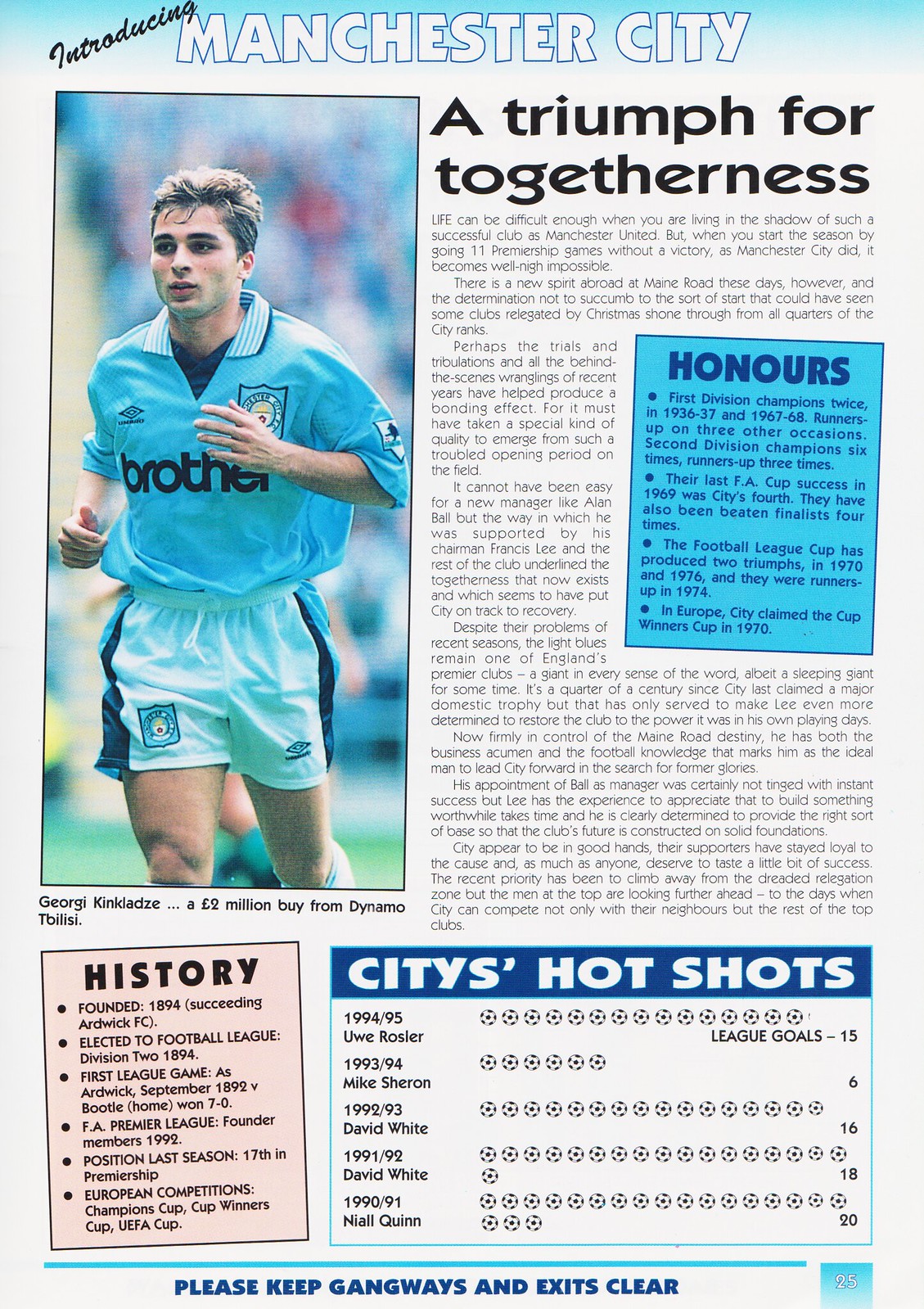This image is likely a scan of a page from a sports program or magazine insert featuring Manchester City Football Club. At the top, a gradient banner transitions from dark blue to white, framing the headline "Introducing Manchester City." Embedded in the upper-left, beneath the gradient, is a photo of a young soccer player identified as George Kinkladze, a £2 million purchase from Dynamo Tbilisi. Kinkladze, a Caucasian male with sandy brown hair, is captured mid-run in blue athletic gear marked with the sponsor "brother." The text to the right of his image, titled "A Triumph for Togetherness," provides an extensive narrative about the club. Halfway through the article, a light blue vertical rectangle with the header "HONOURS" in capital letters lists the club's achievements. Below, a pink box titled "History" details the club's founding in 1894 and initial league election. Adjacent to this, a dark blue bar headlined "City's Hot Shots" outlines player statistics with visuals of soccer balls representing the number of goals per season. The player with the most goals is depicted with 15 soccer ball icons. The page concludes with a notice requesting readers to "Please keep gangways and exits clear."